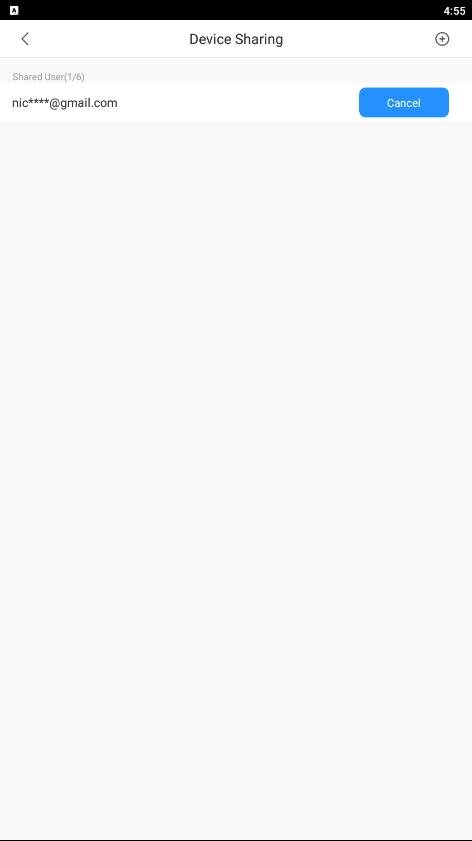This image is a screenshot taken from a mobile phone, capturing a settings page specifically labeled "Device Sharing". The page indicates that there is currently one user sharing the device. The user's email address is partially obscured for privacy, showing as "NIC*****@gmail.com", with four or five asterisks concealing part of the address. On the right-hand side of the screen, there is a blue "Cancel" button, allowing the user to discontinue the device sharing arrangement.

The screenshot was taken at 4:55, as indicated by the time displayed on the device. In the top left corner of the screen, there is a small logo or label, though its details are not clear. The top of the screen features a black rectangle, possibly indicating a status bar, while the bottom of the screen is mostly bare, showing a white background with a thin black line. The image does not display any thumbprint or fingerprint identification areas.